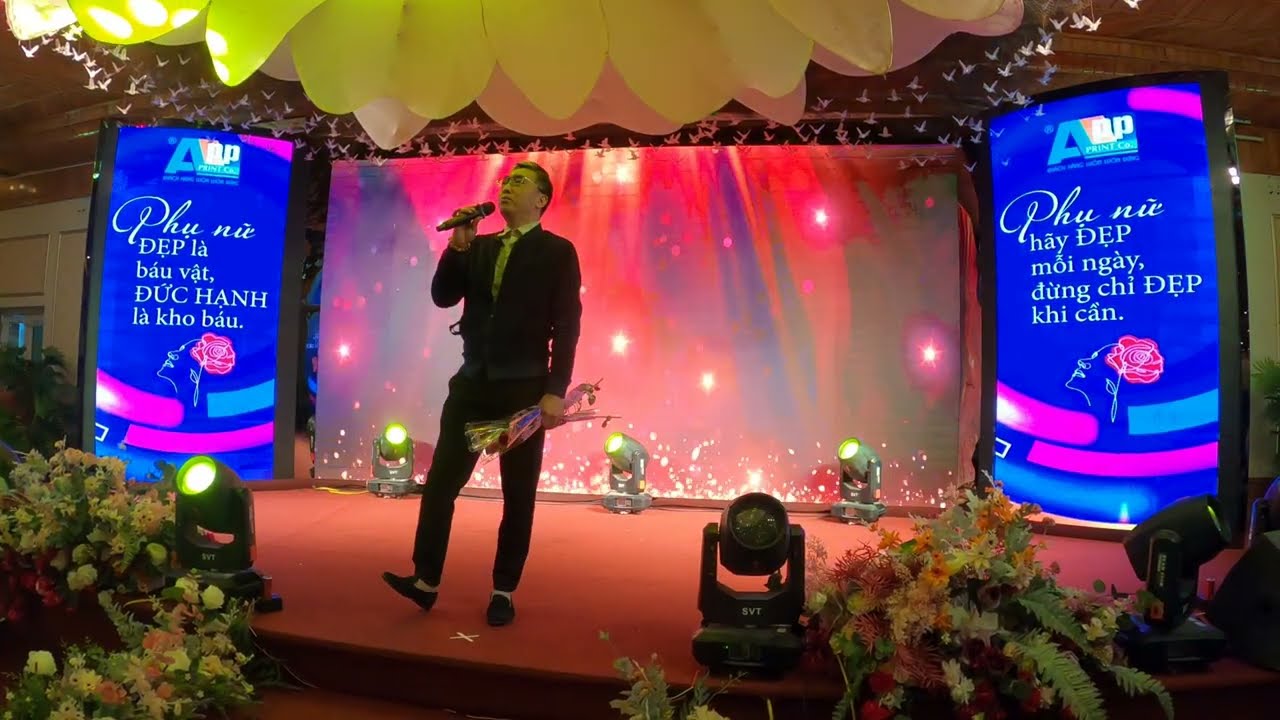This photograph depicts an indoor stage area with a vibrant and colorful setting. The stage has a red carpeted surface and is adorned with artificial flowers scattered across the front part of the stage. Centered on the stage is an Asian man, dressed in a black ensemble that includes a black jacket, black pants, black dress shoes, and what appears to be a colored or gray dress shirt underneath. He is holding a microphone close to his mouth with his right hand, seemingly in the midst of delivering a speech. In his left hand, he holds a bouquet of flowers wrapped in plastic film. The stage lighting includes several spotlights positioned both behind and in front of him. Behind the man, a display screen showcases an array of colors such as red, dark blue, and purple, with decorative elements resembling stars. On the left and right sides of the stage, there are blue rectangular boards featuring text, possibly in Vietnamese, as well as a large yellow flower and paper white birds or doves hanging from the ceiling, adding to the elaborate decorations. The overall ambiance is strikingly vivid and elaborate.